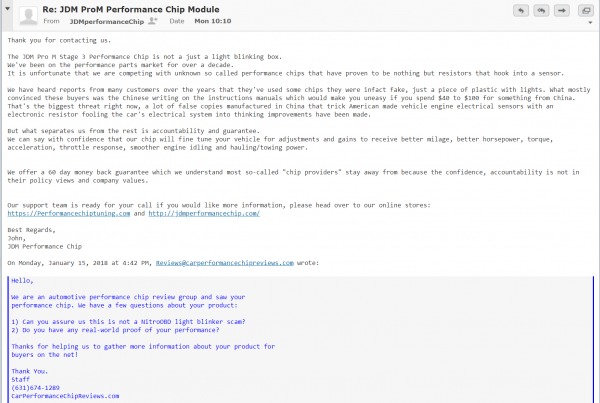**Email Correspondence from JDM Performance Chip Regarding the JDM Pro-M Stage 3 Performance Chip**

**Email Header:**
- **From:** John (JDM Performance Chip)
- **Subject:** Re: JDM Pro-M Performance Chip Module from JDM Performance Chip
- **Date:** Monday, January 15th, 2018 at 4:42 PM

**Email Layout:**
- **Header Bar:** Grey bar at the top containing subject information.
- **Icons (Left to Right):** Person icon, backwards arrow, forwards arrow, files icon, and an indistinct icon resembling a backwards arrow with an additional element.

**Email Content:**
John from JDM Performance Chip responds to an email inquiry:

---

"Dear Reviews Team,

Thank you for contacting us.

The JDM Pro-M Stage 3 Performance Chip is not just a light-blinking box. We've been a prominent figure in the performance parts market for over a decade. Unfortunately, we are currently competing with many unknown so-called "performance chips" that have proven to be nothing more than resistors hooked into a sensor. Numerous customers have reported purchasing fake chips that were merely pieces of plastic with lights, often identified by the Chinese writing on the instruction manuals. It's understandable to feel uneasy after spending $40 to $100 on something from China. This is a significant threat as there are many counterfeit products being manufactured that trick American-made vehicle engine electrical sensors with electronic resistors, falsely indicating improvements.

What distinguishes us from others is our commitment to accountability and guarantee. We proudly assure that our chip can fine-tune your vehicle to achieve better mileage, horsepower, torque, acceleration, throttle response, smooth engine idling, and improved hauling/towing power. We offer a 60-day money-back guarantee, something most so-called chip providers avoid due to their lack of confidence and accountability.

Our support team is available for any inquiries. For further information, please visit our online stores:

- https://performancechiptuning.com
- http://JDMperformance.com

Best regards,
John
JDM Performance Chip

---

**Original Inquiry:**

On Monday, January 15th, 2018, at 4:42 p.m., Reviews at carperformancechipreviews.com wrote:

"Hello, we are an automotive performance chip review group and saw your performance chip. We have a few questions about your product:

1. Can you assure us this is not a Nitro-080 light blinker scam?
2. Do you have any real-world proof of your performance?

Thank you for helping us gather more information about your product for buyers on the internet.

Best,
Staff
(631) 674-1289
carperformancechipreviews.com"